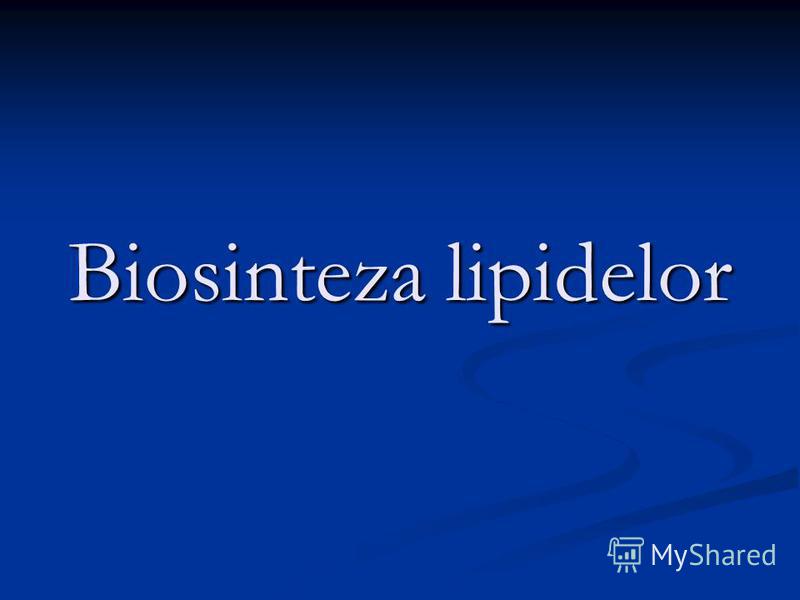The image appears to be a slide from a PowerPoint presentation with a predominantly blue, gradient background that transitions from dark blue to lighter blue as it descends, eventually blending into black at the top. In the center of the slide, the text "Biosintezalipidelor" is prominently displayed in white serif font, with the initial 'B' capitalized. Below this title, there are intricate, squiggly lines that resemble skid marks, rendered in a darker shade of blue against the lighter blue background. In the bottom right corner, the MyShared logo is present, featuring the text "MyShared" in a lighter blue font beside a small, chart-like graphic.